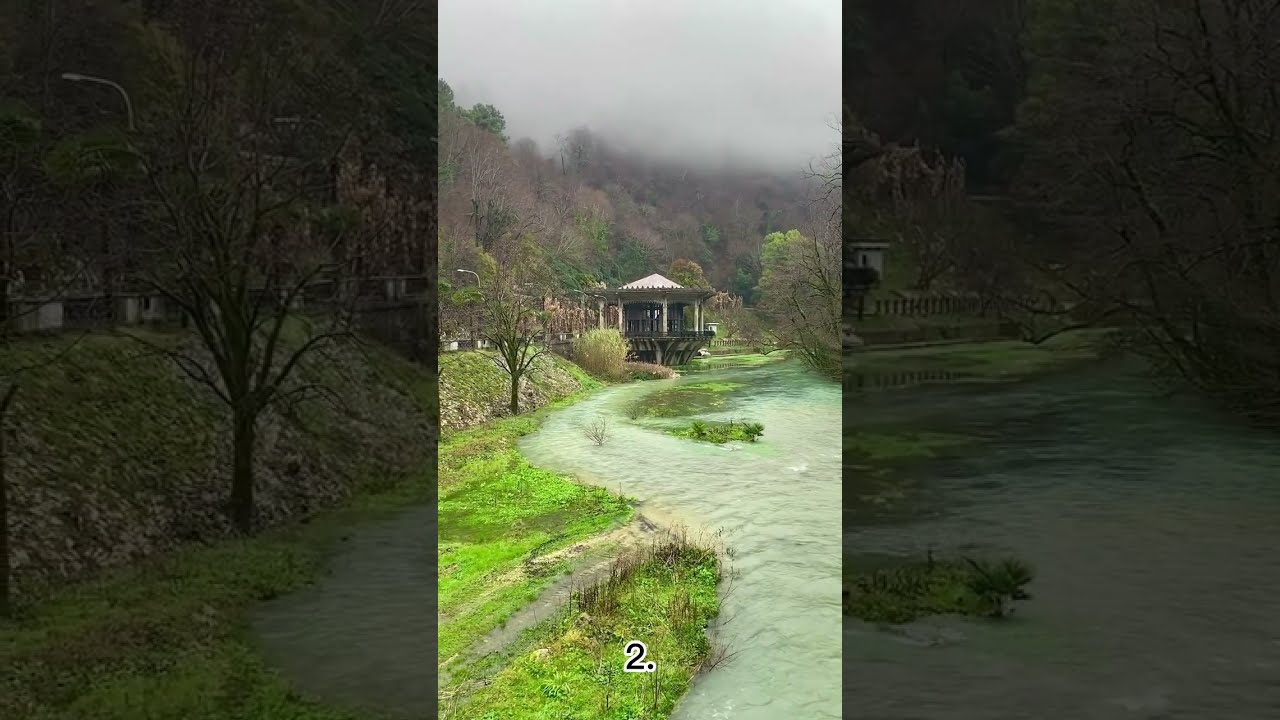The image portrays a serene outdoor scene featuring a quaint gazebo-like structure with a distinctive pyramid-shaped roof and numerous pillars, some of which may be glass. Adjacent to this structure, a creek or small river flows with a striking minty-green hue, occasionally dotted with patches of algae. The waterway is bordered by marshy wetlands and a steep, grassy embankment.

Surrounding the area are a mix of bare deciduous trees and a few that still have green leaves, creating a stark contrast. This is set against a backdrop of a foggy, gray sky, enveloping a hillside that elevates into a mountain range. The overall landscape appears damp and inviting, a picturesque blend of natural elements.

At the bottom-right corner of this scene, a bold number two in black with a white border is superimposed on the image. The lighting across the entire frame is balanced and well-lit, while the edges of the image fade into slightly less illuminated border sections.